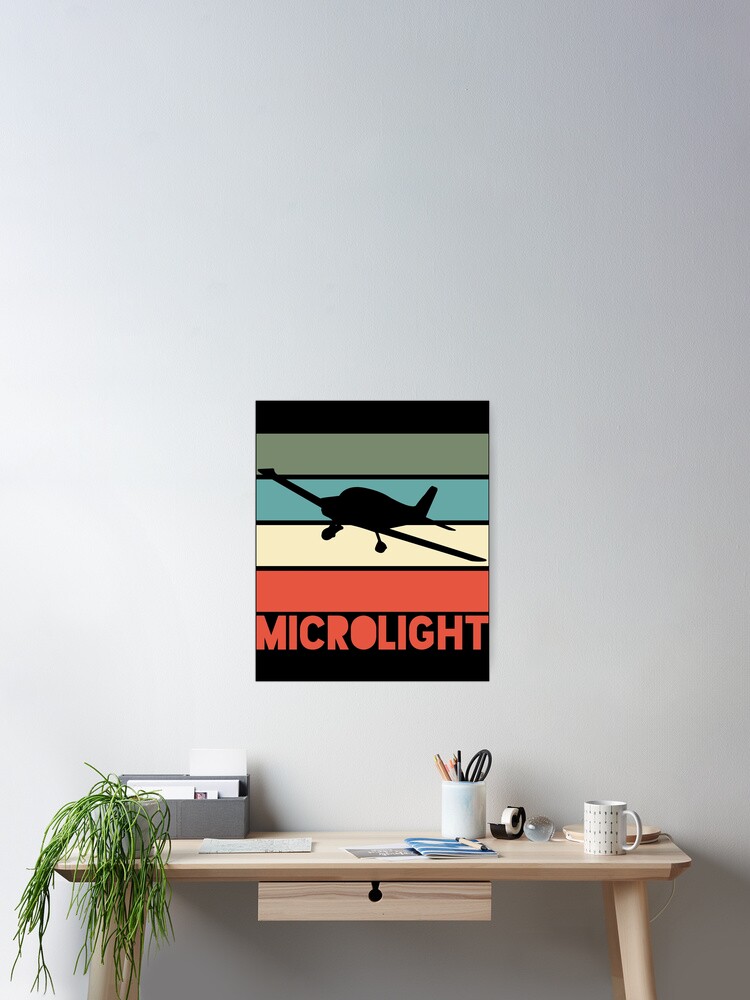The image portrays a minimalist and modern desk setup against a light-colored wall, reminiscent of an IKEA catalog scene. The desk, crafted from light brown wood, features a single drawer and is neatly organized. On the far left, a bright green plant adds a touch of nature, while nearby, an organizer holds scattered pieces of paper and notebooks. Centrally located on the desk, a container holds pencils, pens, and scissors, accompanied by a roll of tape. To the right, a sleek white coffee mug sits beside a contemporary white table lamp extending its arm to illuminate the workspace. Above the desk, a vibrant poster with the word "Microlight" prominently displayed captures attention. The poster showcases an airplane silhouette amidst horizontal stripes in a spectrum of colors including black, green, blue, white, orange, olive green, and yellow. The overall setup is clean and functional, blending practicality with aesthetic appeal.